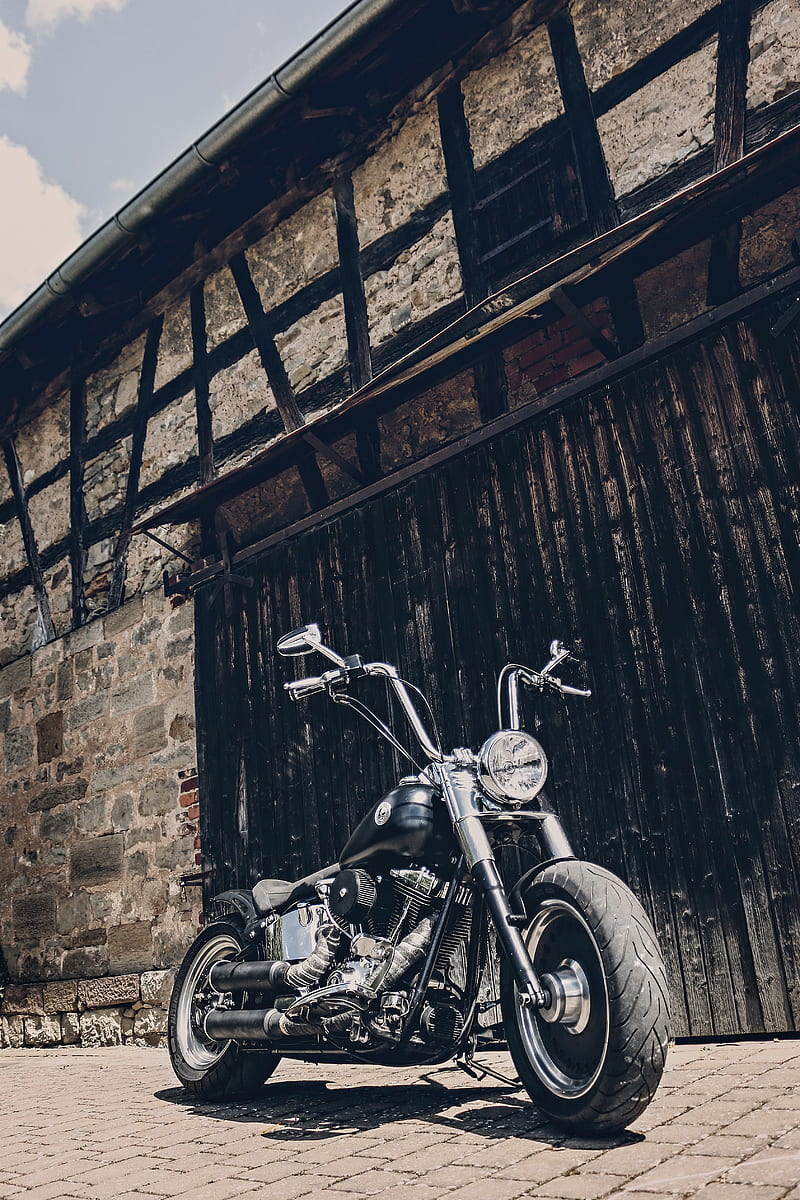In this outdoor photograph, we see a stylish black motorcycle with wide tires parked on a light brown, rectangular brick-paved street. The motorcycle's design is accentuated by its prominent chrome elements, clear headlight, and silver handlebars. The background features a building structure, resembling an old barn, with a mixed composition of brick and concrete materials. A large black, somewhat metallic, door is noticeable toward the middle right side of the structure. The building also showcases black stripes that are not perfectly vertical. Above the building, the sky is predominantly gray with patches of white clouds. Sunlight illuminates the scene, casting the motorcycle's shadow onto the ground, adding to the overall detailed and textured appearance of the photograph.